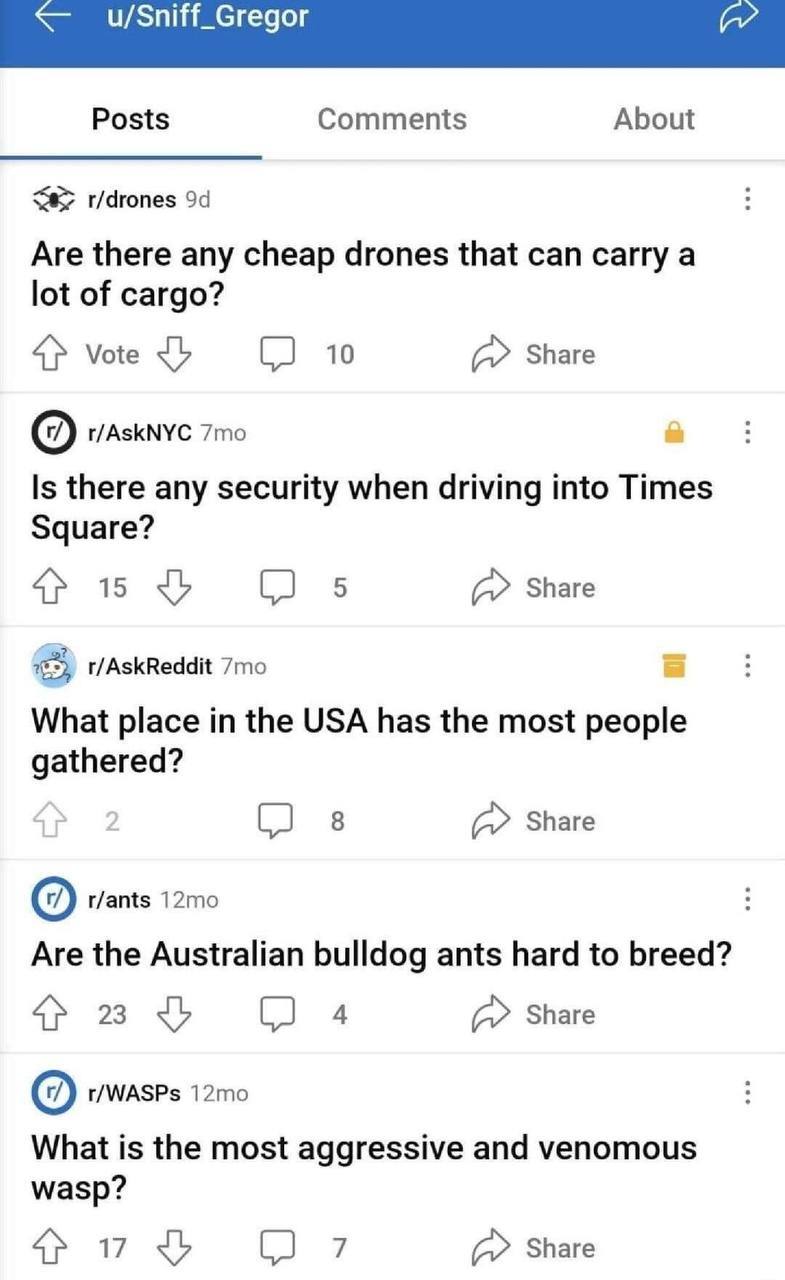The image depicts a tall and narrow screenshot of a Reddit user's account, specifically the profile of u/sniff_Gregor. The top 5-10% of the image features a blue background with a white left arrow and the username "u/sniff_Gregor" written in white text. Below this header, the profile interface is visible, showcasing three navigation tabs: "Posts," "Comments," and "About," with "Posts" highlighted in bold with a blue underline indicating it is selected.

The image portrays several posts under the "Posts" tab. The first post, made in the r/drones subreddit nine days ago, asks in black text, "Are there any cheap drones that can carry a lot of cargo?" The second post, seven months ago in the r/AskNYC subreddit, inquires, "Is there any security when driving into Times Square?" The third, in the r/AskReddit subreddit, questions, "What place in the USA has the most people gathered?" The fourth post, found in the r/ants subreddit, asks, "Are the Australian bulldog ants hard to breed?" Finally, the fifth post from twelve months ago in the r/wasps subreddit, queries, "What is the most aggressive and venomous wasp?" This last post has garnered 17 upvotes and seven comments.